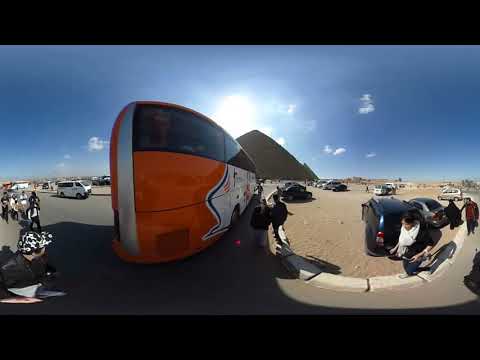In this bright daytime image, a bustling outdoor scene in Egypt is vividly captured, with the iconic silhouette of a pyramid standing tall in the background under a mostly blue sky adorned with minimal white clouds. Dominating the center of the image is a large, red and white two-story tour bus, indicative of a popular tourist attraction for viewing the pyramids. The setting is lively with numerous tourists, many dressed in jackets and hats, walking around the paved, gray road and gravel areas. The sun shines brightly, casting an impressive glow over the pyramid. Surrounding the bus are several parked vehicles, including a blue SUV and a gray car, with more cars visible in the distance. The surrounding area is characterized by curbside rocks cut into rectangles and scattered small trees, adding to the environment's dynamic and scenic nature.